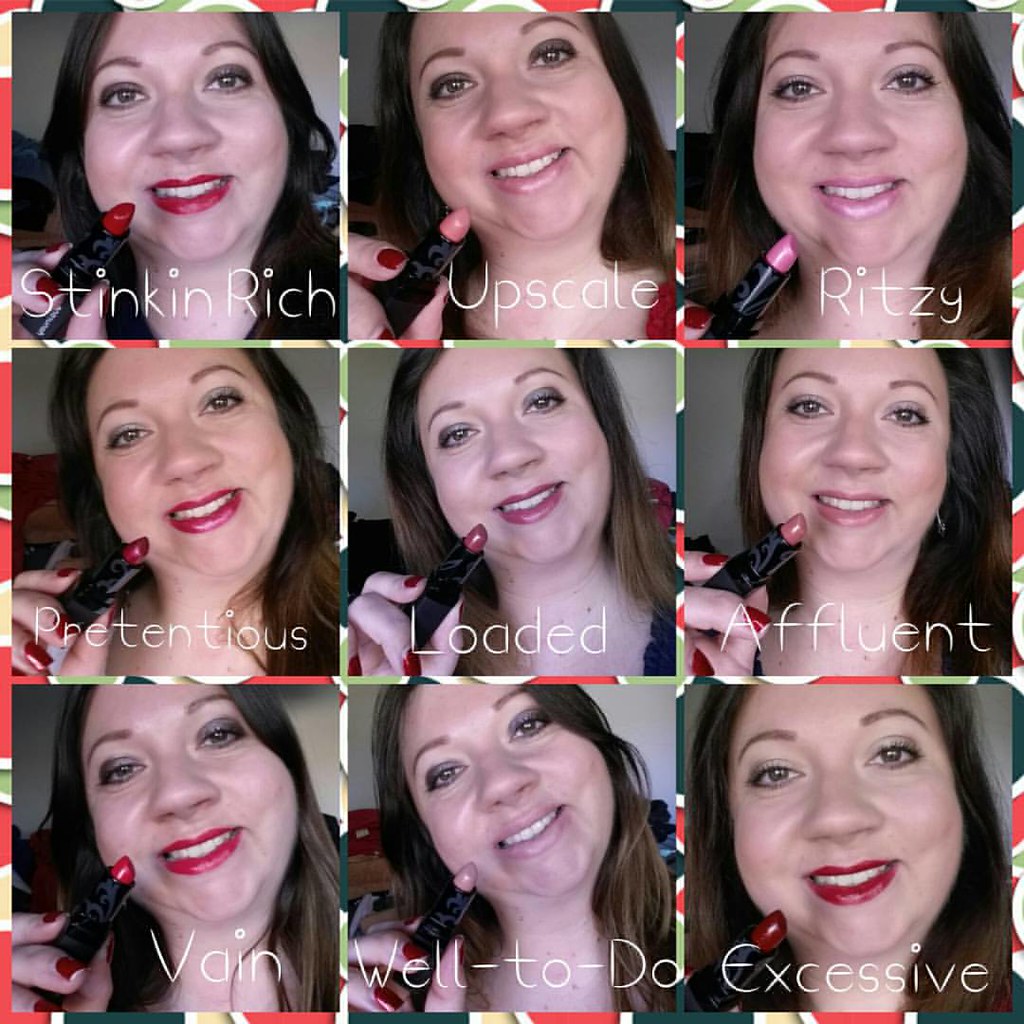In this captivating image often seen on Instagram or Facebook, a makeup influencer showcases nine different lipstick shades in a 3x3 grid format. The image features the head and decollete of the same woman, posed identically in each square to emphasize the variety of lip colors. Each square has a caption in white letters at the bottom, linking each lipstick shade to phrases representing wealth and style. The shades are Stinking Rich, Upscale, Ritzy, Pretentious, Loaded, Affluent, Vain, Well-to-Do, and Excessive. The colors range from extremely bright, like Stinking Rich, Pretentious, and Excessive, to very subtle, such as Well-to-Do. These captions and colors suggest a playful commentary on the concept of wealth and its various depictions. The overall image is bordered with a small, colorful flower pattern in reds, greens, yellows, and whites, adding a decorative touch to the ensemble. This visually engaging display combines aesthetic beauty with a whimsical take on luxury through lipstick choices.